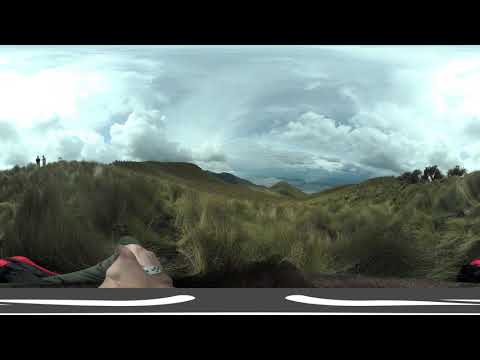The image depicts a vast outdoor scene characterized by a rolling grassy hill adorned with green trees. The landscape is blanketed under a sky densely packed with puffy white clouds, casting an overcast mood, with patches of dark blue peeking through the cloud cover. 

On the top-left side of the hill, two indistinct figures stand, looking distant and almost silhouetted against the cloudy backdrop. The bottom part of the image reveals a gray asphalt road with white arrows pointing in opposite directions, hinting at a crossroads. Additionally, an indistinguishable object sits at the very bottom of the image.

The scene feels expansive, possibly taken with a 360 panorama, giving a slightly distorted view that makes it look like the observer is atop the hill. In the foreground, there appears to be another person, possibly wearing a ring, walking towards the figures on the hill. The overall setting is natural, evoking a serene yet slightly mysterious atmosphere typical of a cloudy day in a wide-open grassy area.